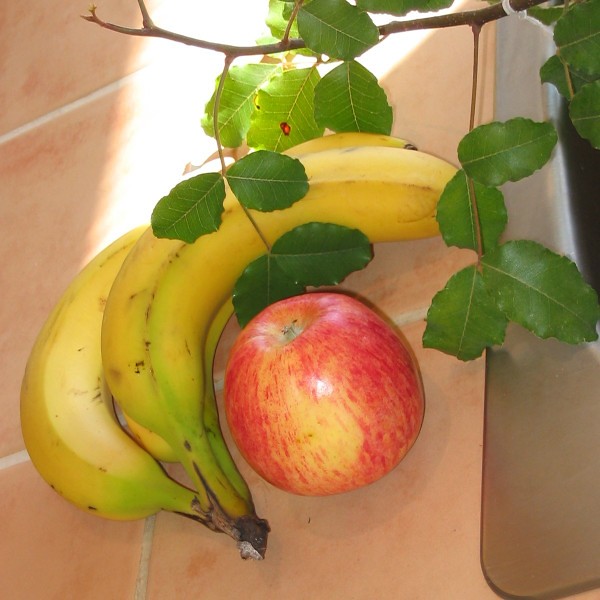A close-up image captures an assortment of fruit and foliage in rich detail. The focal point features three bananas with vibrant yellow skins, accented by green tips where they cluster together; minor brown spots suggest they are perfectly ripe. Nestled beside the bananas is a radiant apple, its skin a blend of deep red and warm yellow patches, reminiscent of a Gala apple. The apple's surface gleams with reflected light, highlighting its smooth texture and the tiny stem at its crown.

All the fruit rests on a rustic terracotta tile countertop with a raw, unglazed finish, adding an earthy backdrop to the vibrant produce. Overhanging the fruit is a tree branch adorned with several leaves, some of which are sunlit, displaying intricate vein patterns. A ladybug perches on one of the leaves, adding a touch of natural whimsy. The sunlight filters through a nearby window, casting angular light patterns that intersect the scene. A white string is tied around the branch, suggesting a deliberate arrangement or support, completing the picturesque composition.